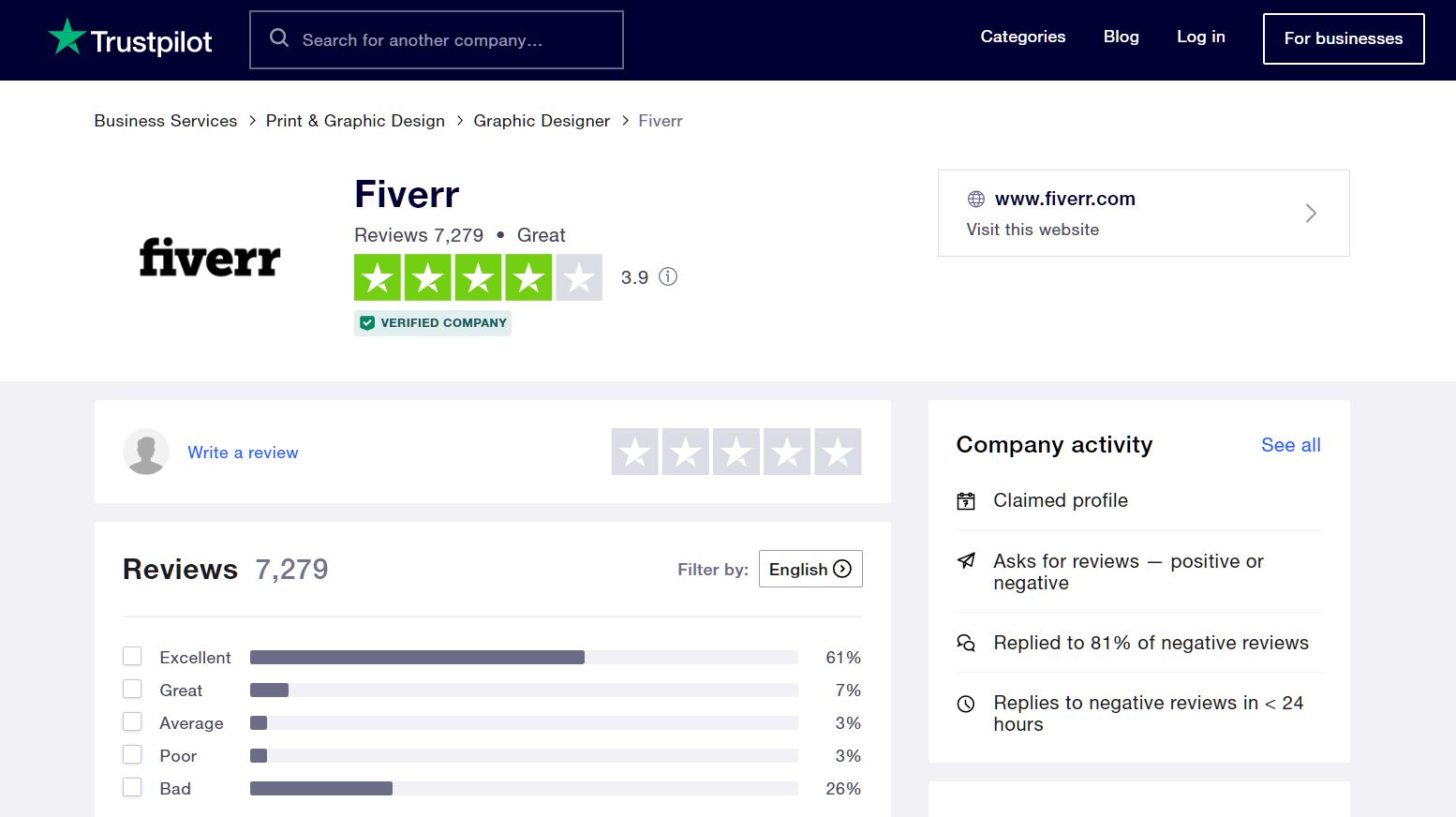This image captures a review section from the Trustpilot website, which is identified by its logo in the top left corner, featuring "Trustpilot" written in white letters accompanied by a green star. The specific webpage displayed rates the online marketplace Fiverr, denoted by its name "Fiverr" prominently written in bold letters.

Adjacent to the Fiverr name, there is a star rating system available, where users can rate their experience out of five stars. In this instance, four out of the five stars are filled in green, indicating a rating of 3.9. This rating is based on a substantial number of reviews—7,279 to be exact. Trustpilot offers a breakdown of these reviews: 61% of users rated Fiverr as 'Excellent,' 7% as 'Great,' 3% as 'Average,' 3% as 'Poor,' and 26% as 'Bad.'

On the sidebar to the right, there are details about company activity. Notably, Fiverr has a claimed profile, actively asks for reviews whether positive or negative, and responds to 81% of the negative reviews. Furthermore, it mentions that Fiverr typically replies to negative reviews in less than 24 hours, highlighting their commitment to customer feedback.